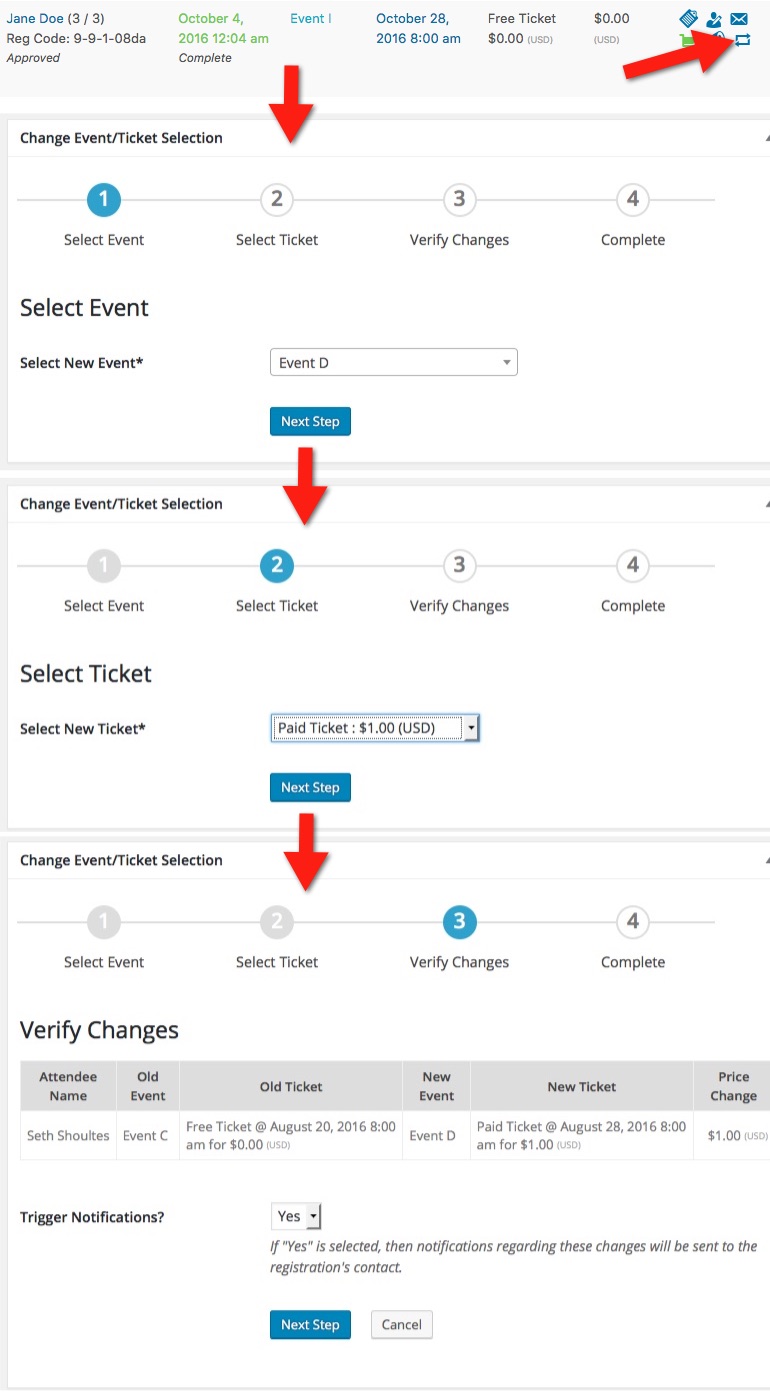**Image Description: Event and Ticket Selection Interface**

The image displays an interface for changing event and ticket selections. At the top, it shows the user Jane Doe, indicating this is screenshot 3 of 3 with Jane's registration code labeled as 9-9-1-08DA, and it is approved. Below this, the date October 4, 2016, 12:04 AM is listed as complete.

**Section Breakdown:**

1. **Event Details:**
   - **Event 1:** Scheduled for October 28, 2016, at 8:00 AM. The current ticket is free ($0).
   - **Navigation Arrows:** One arrow points to the right and another arrow points downward from Event 1.

2. **Change Event/Ticket Selection Interface:**
   - **Options:** 
     - Select Event 1
     - Select Ticket 2
     - Verify Change is Complete

3. **Event Selection and Dropdown:**
   - **Select Event:** Options available from a dropdown menu labeled as Event D.
   - **Next Step:** Indicated by an arrow pointing down.

4. **Ticket Selection Interface:**
   - **Select Ticket:** 
     - Select New Ticket from a dropdown menu
     - Available option: Paid Ticket ($1 USD)
   - **Next Step:** Arrow pointing downward to indicate another step.

5. **Verification Section:**
   - **Current Selection Details:** 
     - Verify Changes shows as selected
     - Attendee: Seth Sheltz
     - Old Event: Event C with a Free Ticket on August 20, 2016, at 8:00 AM ($0 USD)
     - New Event: Event D with a Paid Ticket on August 28, 2016, at 8:00 AM ($1 USD)
   - **Trigger Notification:** Yes/No option appears for sending notifications regarding these changes to the registration's contact.

**Bottom Buttons:**
- **Next Step:** A blue box with white writing
- **Cancel:** A white box with gray writing